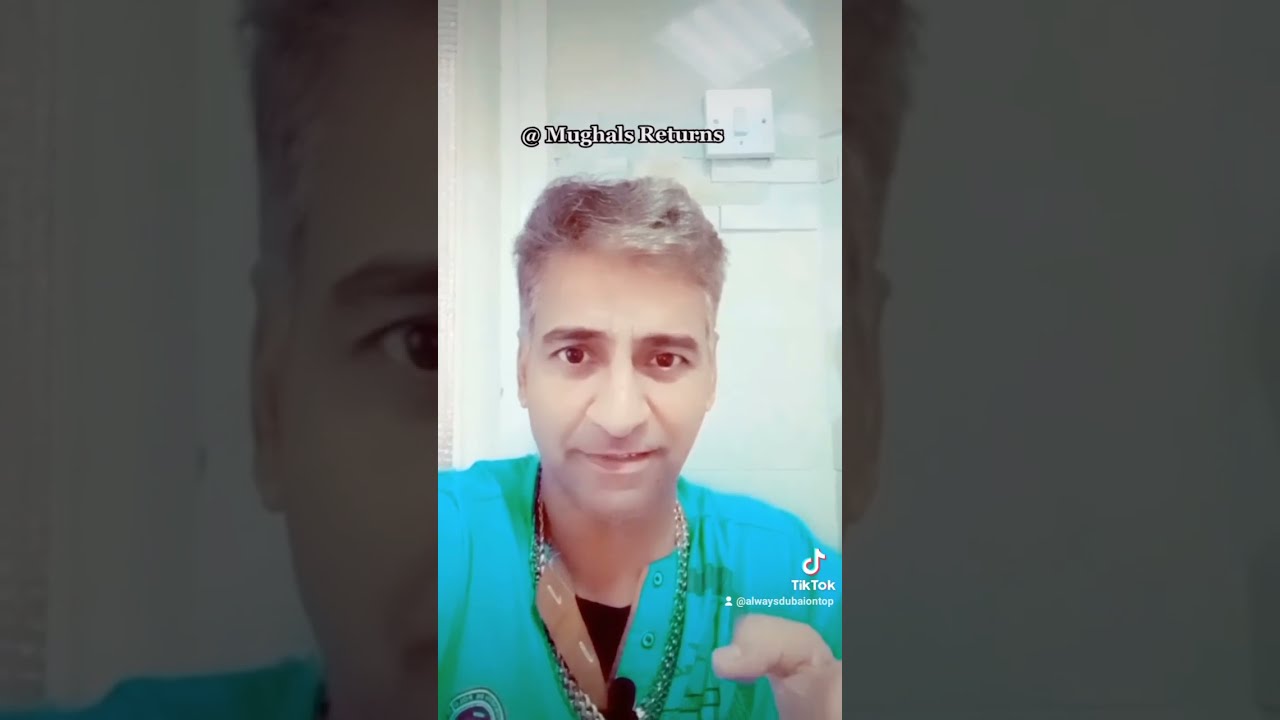The image features a man seated and facing the camera with a direct gaze. He sports wavy, grayish-silver hair mixed with dark strands, and a faint smile. He is wearing a turquoise button-up shirt with green designs, the top two or three buttons undone, revealing a black t-shirt underneath. Around his neck hangs a long, gold and silver chain that disappears out of the camera's frame. The background is a stark white wall with indistinct white objects affixed to it. The image bears the TikTok logo and a username at the bottom right, indicating its origin from the TikTok platform. Above the man's head reads "@MughalsReturns," suggesting possible advertising content. The image is divided into three panels; the central panel, containing the main photograph, constitutes about a quarter of the image's total horizontal width. The left and right panels are darker and consist of blown-up, grayed-out segments of the central photo. The man’s left hand is visible in the foreground, thumb facing towards the camera, adding an engaging dynamic to the image.